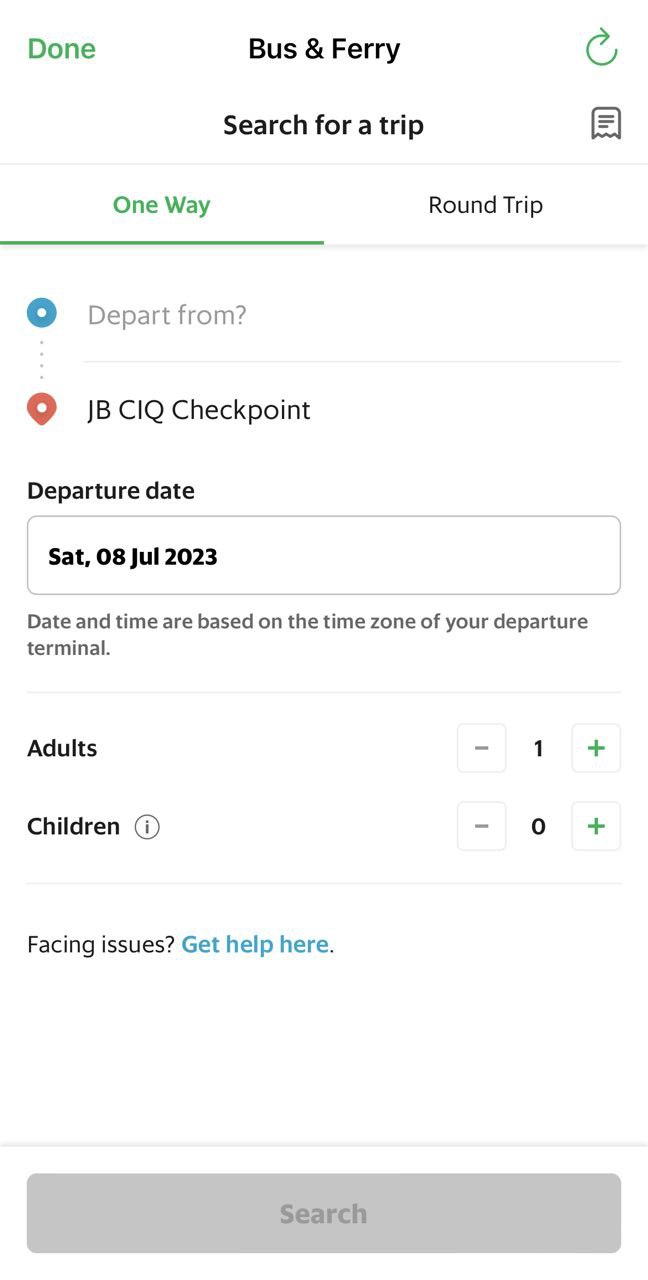The image appears to be a screenshot from a mobile application used for booking a bus and ferry trip. At the top of the interface, there is a header labeled "Bus and Ferry" with an option to "Search for a Trip." The user can select either a one-way trip or a round trip. The next section prompts the user to input their departure location, which is currently set to "JBCIQ checkpoint," though the meaning of this term is unclear.

The user can then select their departure date; in this example, the date chosen is Saturday, 08 July 2023, with a note indicating that the date and time are based on the time zone of the departure terminal. Below this, there is an area where the user can select the number of travelers, with the current selection being one adult and no children.

At the bottom of the screen, there is a light blue link stating, "Facing issues? Get help here," which likely directs users to a support page. At the top right corner, there is a "Done" button that users can click once they have completed their selections. Finally, at the bottom of the interface, there is a prominent "Search" bar, which presumably allows users to look for available bus and ferry trips based on the entered criteria.